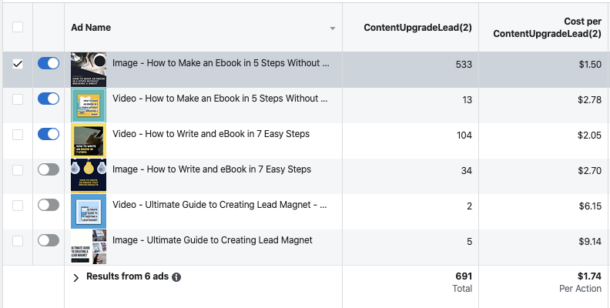The image is a screenshot from what appears to be an e-book or audiobook-related website, with a predominantly white background at the top. At the top, there's a drop-down menu explaining the sections. On the far left, there's an unselected checkbox labeled "Select All." To its right is another option labeled "Add Name," which features a small drop-down arrow.

Beneath this, the text reads "Content Upgrade Lead (2)" followed by "Cost Per Content Upgrade Lead (2)." Further down to the left, there are six options displayed in a list. The first item in the list is checked, and the first three options have active (blue) radio buttons. The remaining three options are indicated as inactive by gray radio buttons.

Following these selection options, the display includes six rectangular image/video thumbnails with associated text and cost details for various ad content. The items are listed as follows:

1. Image titled "How to Make an E-book in Five Steps Without" priced at $533.50.
2. Video titled "How to Make an E-book in Five Steps Without" with two price points: $13.00 and $2.78.
3. Video titled "How to Write an E-book in Seven Easy Steps" priced at $104.00 and $2.05.
4. Image titled "How to Write an E-book in Seven Easy Steps" priced at $34.00 and $2.70.
5. Video titled "Ultimate Guide to Creating Lead Magnet" priced at $2.00 and $6.15.
6. Image titled "Ultimate Guide to Creating Lead Magnet" priced at $5.00 and $9.14.

At the bottom, the summary of the data reads: "Results from six ads, $691.00 total, $1.74 per action."